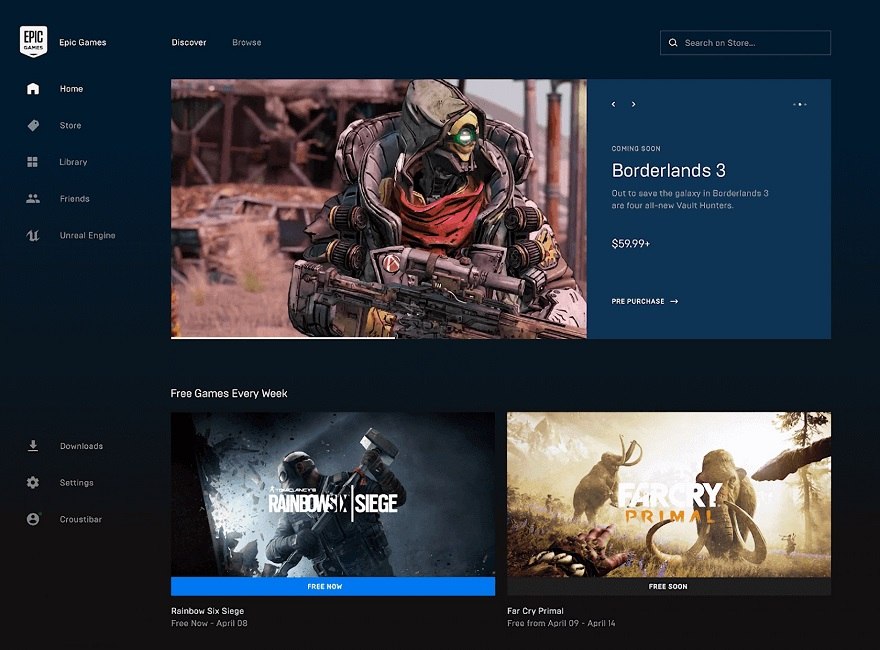The image showcases a dark navy blue background, prominently featuring the Epic Games logo at the top, which is an inverted white pentagon with the name "Epic Games" written in blue. Below the logo, the white text lists various sections including Home, Store, Library, Friends, Unreal Engine, Download Settings, and an unfamiliar term "C-R-O-U-S-T-I-B-A-R."

At the very top, the navigation bar displays options such as Discover, Browse, and a Search Box with the prompt "Search on Store..."

The main focus of the display is on three games. The topmost game appears to feature an alien robot holding a gun, labeled "Coming Soon, Borderlands 3: How to Save the Galaxy in Borderlands 3." The price for this game is listed as $59.99, with an option to pre-purchase indicated by an arrow pointing right.

Below to the left, an advertisement highlights "free games every week," featuring a character equipped with a mask and a sledgehammer, labeled "Rainbow Six Sledge." The text "Free Now" suggests that "Rainbow Six Siege" is available for free until April 8. 

Next to this, the image promotes "Far Cry Primal," marked by an orange-and-white title and featuring images of two mammoths. This game is also advertised in the free zone.